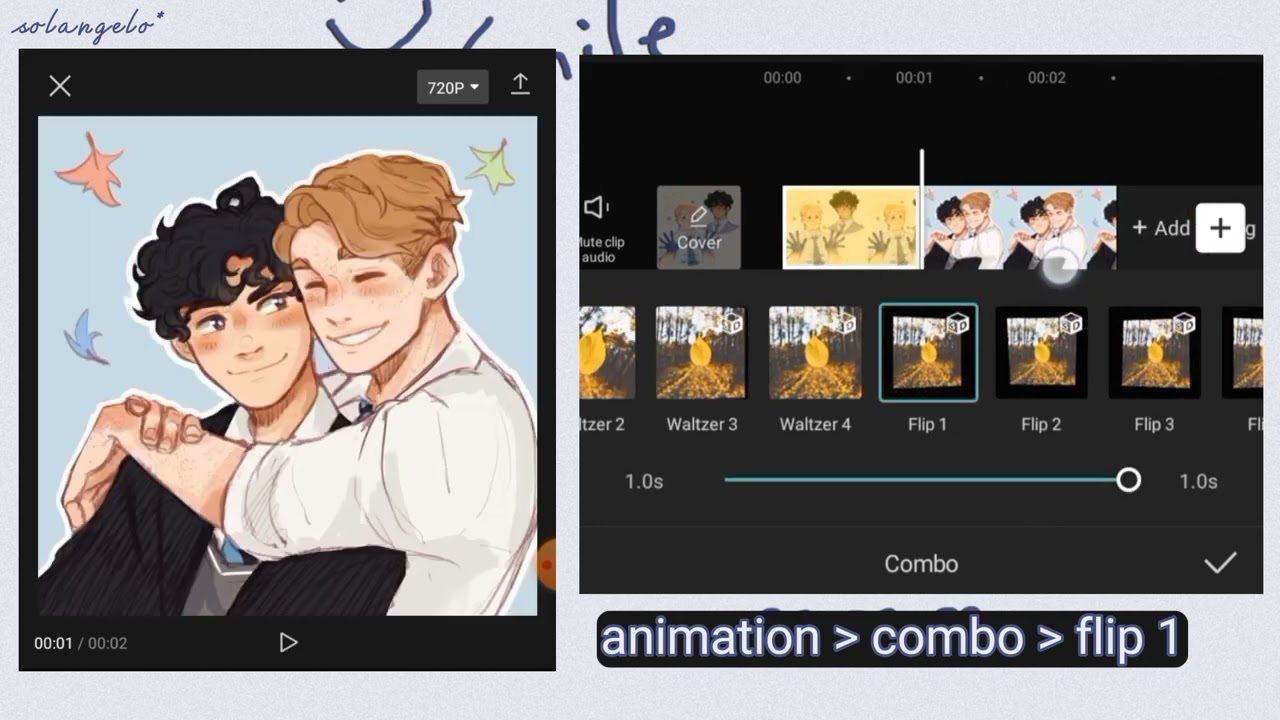A detailed wide screenshot captures a video editing software interface at the moment of active use. The primary focus on the left side of the screen features an intimate photograph of two young men sitting closely together, suggesting a tender, possibly romantic relationship. The man in the foreground, with black hair, is enveloped in the arms of his companion, who has blonde hair. This affectionate pose underscores a genuine connection between the two, hinting at more than mere friendship.

On the right side, the editing software is prominently displayed, focusing on a two-minute video clip currently under modification. The timeline at the bottom of the screen is segmented into individual frames, each clearly visible, indicating meticulous frame-by-frame adjustments. The playhead is positioned at the middle frame, suggesting that the editor is fine-tuning this specific moment of the clip. Various editing tools and options are visible, emphasizing the detailed work being done to either enhance the visual quality or trim the video. The combined imagery of personal connection and technical precision provides a rich narrative of storytelling through visual and emotional lenses.